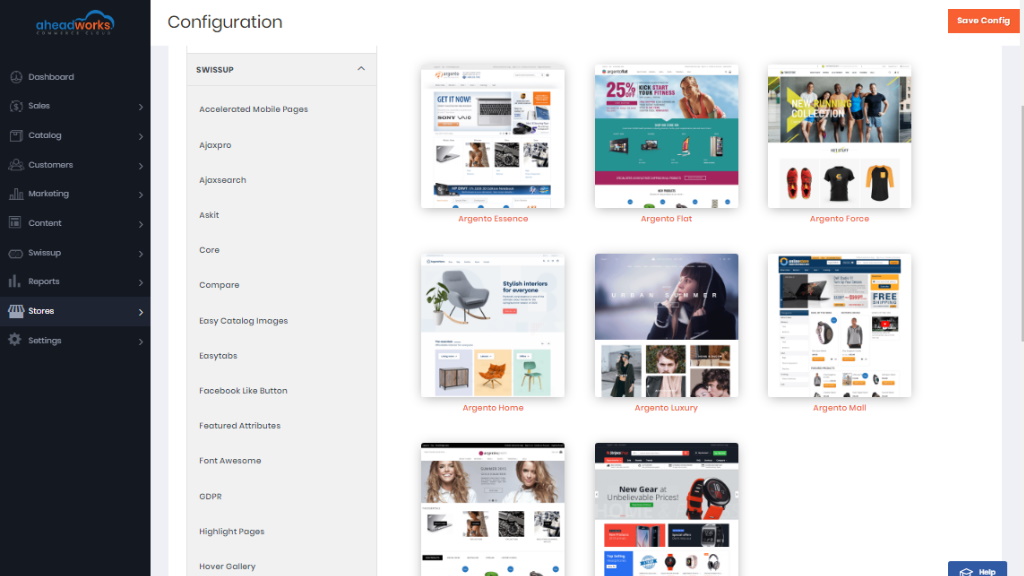This image depicts a configuration page from the AHEADWORKS application or website. The design is predominantly white, with a dark blue or black pane along the left side. At the top of this pane, the AHEADWORKS logo is displayed in blue and orange. Below the logo, a navigational menu lists options including Dashboard, Sales, Catalog, Customers, Marketing, Content, SWISUP, Reports, and Stores, with the "Stores" option currently highlighted. Beneath the menu, there is a settings button.

The central area of the page, which has a white background, features various images showcasing different design options. A gray pane labeled "SWISUP" lists numerous tools and features such as Accelerated Mobile Pages, AJAX Pro, AJAX Search, ASKIT Core, Compare, Easy Catalog Images, Easy Tabs, Facebook Like Button, Featured Attributes, Font Awesome, GDPR, Highlight Badges, Pages, and Hover Gallery. To the right of this pane, several style options are displayed, specifically Argento Essence, Argento Flat, Argento Force, Argento Home, Argento Luxury, and Argento Mall.

At the upper right corner of the page, there is an orange button labeled "Save Config," and at the lower right corner, a blue button labeled "Help." The overall layout suggests this is a configuration page where users can customize various aspects of the AHEADWORKS application or website, reviewing and applying different styles and settings.